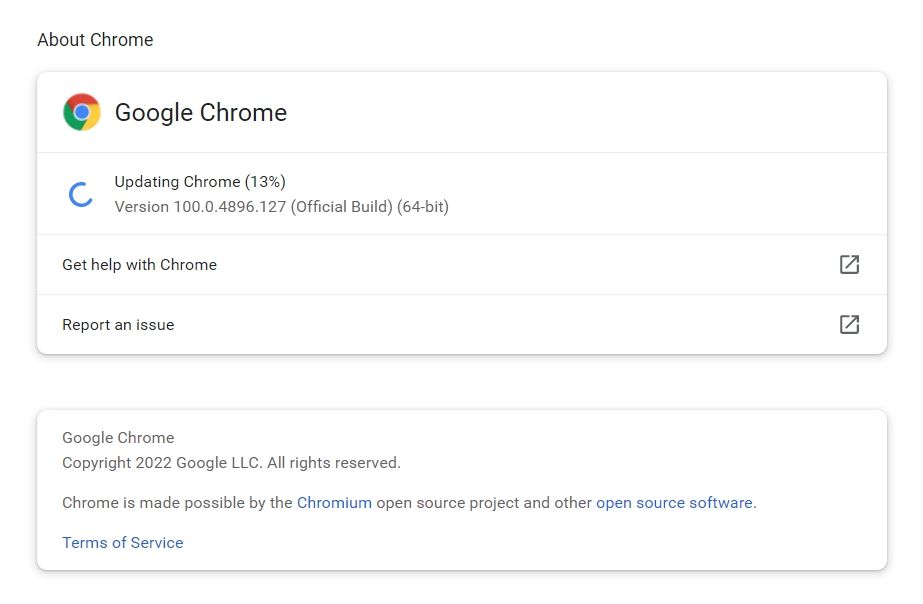This image captures a digitally rendered section of the Google Chrome browser. At the top, a prominent rectangular header displays "Google Chrome" alongside the recognizable Chrome icon, resembling a colorful ball with a blue center surrounded by red, green, and yellow segments. Below this header, the status "Updating Chrome 13%" is shown, accompanied by a circular progress bar where 13% is filled in blue, indicating the update progress.

Further down, the section includes links for "Get help with Chrome" and "Report an issue." The footer of the image provides copyright information stating "Google Chrome © 2022, Google LLC. All rights reserved." Accompanying this is a note that reads, "Chrome is made possible by the Chromium open-source project and other open-source software." Key phrases such as "Chromium" and "open-source software" are highlighted in blue, distinguishing them from the predominantly gray-black text. At the very bottom, another clickable blue link labeled "Terms of Service" invites users to view additional information.